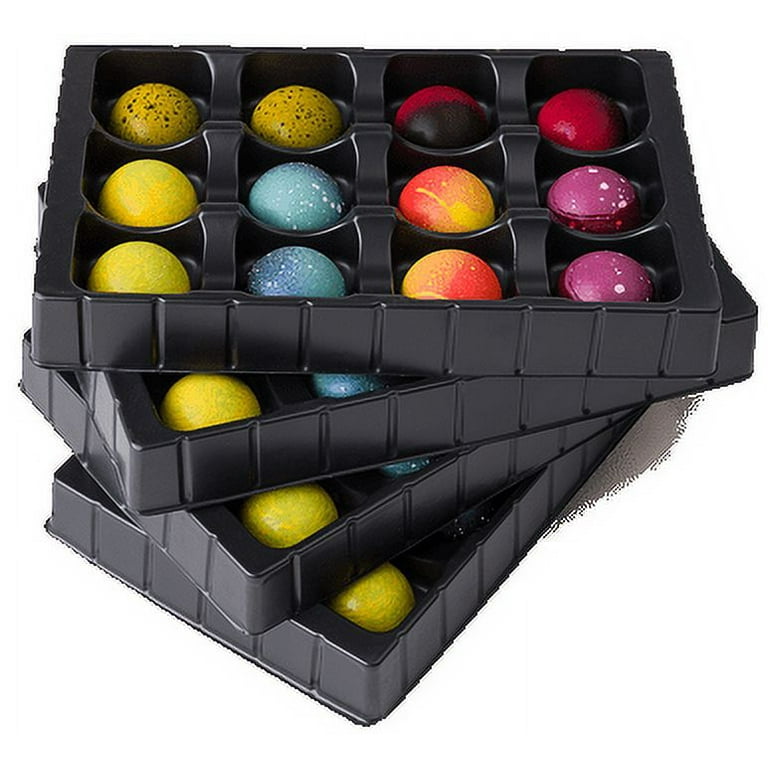The image depicts four black trays, each with 12 compartments arranged in three rows of four, containing round objects that appear to be candies. The trays are slightly fanned out, revealing at least one ball in each of the trays underneath the top one. The balls in the compartments vary in color and pattern. In the top tray, the arrangement includes two yellow balls with multicolored speckles, two solid yellow balls, two balls that are half black and half red, two blue balls with white speckles, two red and yellow tie-dye balls, and two purple balls with white speckles. The overall color palette transitions from yellows on the left to blues, reds, and purples on the right. Each tray contains a consistent color arrangement, with the balls appearing edible due to their candy-like appearance.